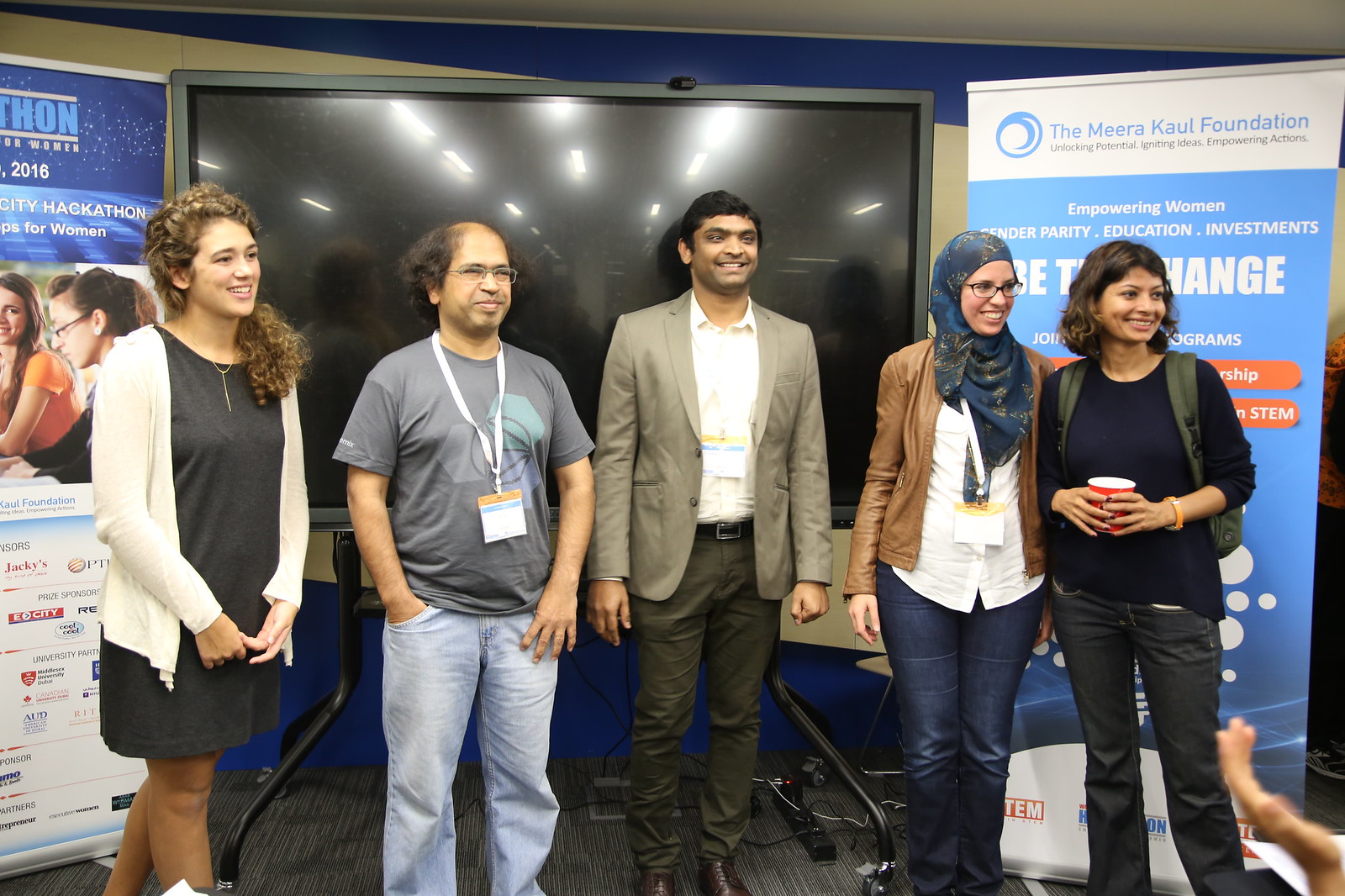In this color photograph, five people stand side by side at the front of a room, seemingly participating in a convention or conference. They are all facing and smiling toward someone or something off to the right side of the image. The group is composed of three women and two men. Starting from the left, the first individual is a young woman with long, curly dark hair, dressed in a short black dress paired with a white cardigan. Next to her, a man with a receding hairline and wire-rimmed glasses is wearing a gray t-shirt and blue jeans. The central figure, a young man, is dressed in a beige blazer, brown pants, and a white shirt. On his right is a woman in a brown blazer over a white shirt and blue jeans, adorned with a blue headscarf. The last person, on the far right, is a young woman in a dark shirt, blue jeans, and an olive vest, holding a red cup of beverage. 

Each person wears a lanyard around their neck, indicating their participation in the event. Behind them, a large TV monitor takes center stage, flanked by two pull-up banners. The banner on the left and right features text associated with the "Miracle Foundation," which aims to empower women, achieve gender parity, foster education, and encourage investments. The colors in the image range from the diverse attire of the people—light blue, gray, tan, white, brown, and black—to the red of the cup and the orange, white, and blue hues of the banners. The setting conveys a professional and collaborative atmosphere, likely reflecting a presentation or discussion aimed at unlocking potential and igniting ideas.